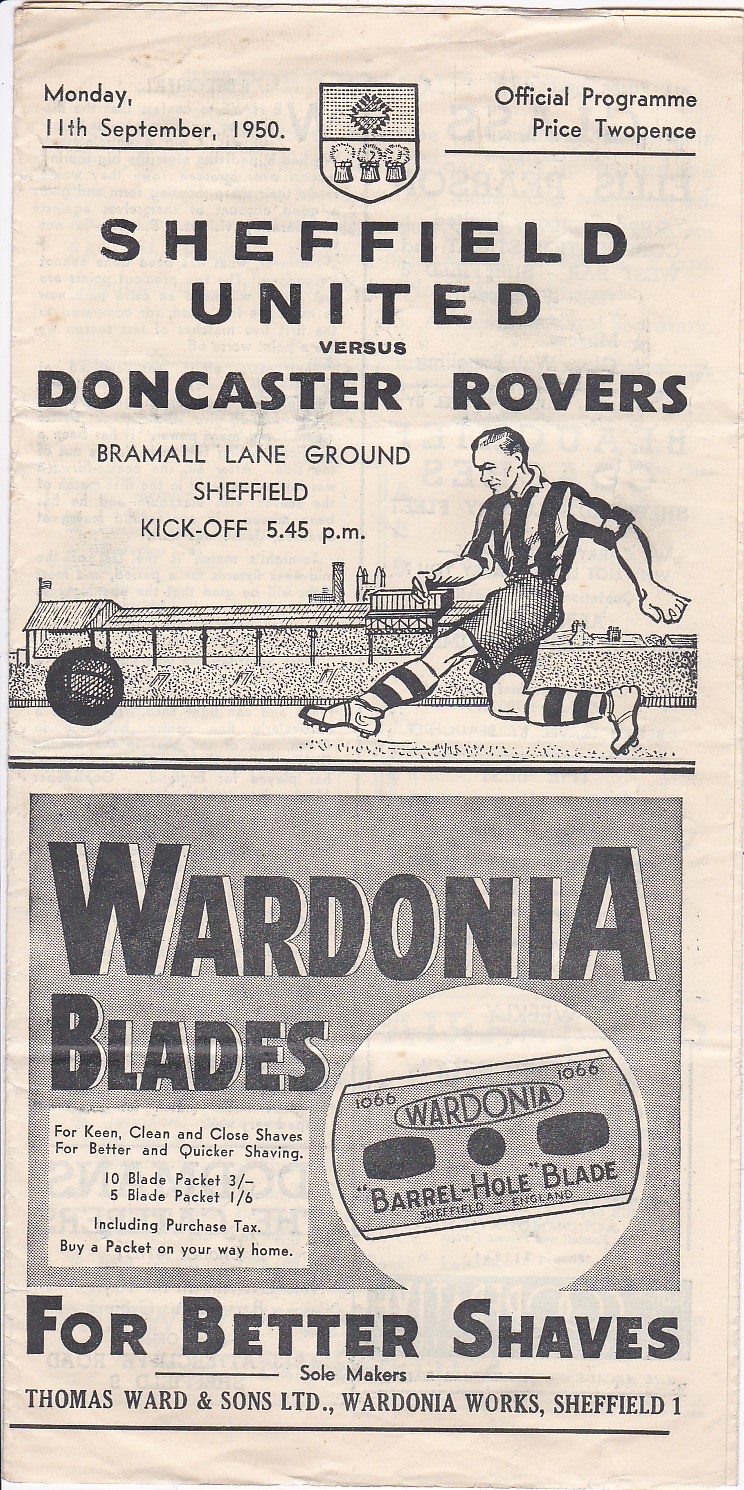This image is an aged, black and white newspaper front page, dated Monday, 11th September 1950, featuring the official program for a soccer match between Sheffield United and Doncaster Rovers. The masthead includes a centrally placed shield, dividing into two sections: the top with a diamond and the bottom depicting three bushels of hay. Below the shield, bold text announces the match details, including the location, Bramall Lane Ground, Sheffield, and the kickoff time of 5:45 p.m. An illustration captures a soccer player mid-kick in front of stylized stadium stands. The lower portion of the newspaper transitions into an advertisement for Wardonia Blades, extolling their benefits for keen, clean, and close shaves. The ad details prices for 10-blade and 5-blade packets, inclusive of purchase tax, and introduces the Wardonia Barrel Hole Blade, manufactured by Thomas Ward and Sons, LTD, at Wardonia Works, Sheffield 1. The page's overall aesthetics convey a faded, yellowing appearance, typical of old newspapers.